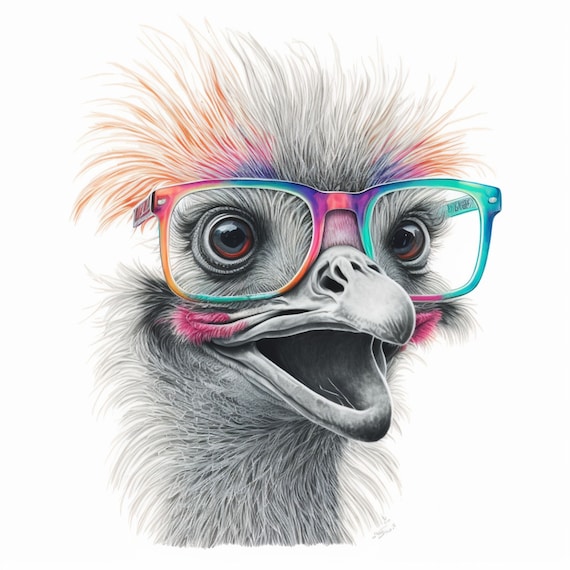The image is a detailed, digitally drawn illustration of an ostrich with a striking combination of realistic elements and imaginative coloring. The focal point is the ostrich, which is predominantly black, white, and gray. The ostrich is adorned with multicolored glasses that stand out against its more muted tones. The glasses feature a blend of green, purple, pink, blue, orange, yellow, and aquamarine hues, adding a vibrant splash to the artwork. 

The ostrich's eyes are gray with hints of black and red, giving them a piercing, almost surprised expression. The creature's beak, prominently displayed with four nostril holes, is open, revealing the inside of its mouth. Surrounding the beak and mouth area is a subtle touch of pink. The ostrich's feathers are intricately drawn, with the head showcasing a mix of colors: primarily black and white, but also featuring patches of peach, pink, purple, red, and orange. 

Despite the vibrant glasses and multicolored plumage, the background remains a simple, stark white, emphasizing the ostrich’s detailed and vibrant depiction. The overall composition of the drawing suggests the ostrich is outdoors, and it appears to be looking towards the bottom right-hand corner of the image, adding a dynamic sense of depth and perspective to the artwork.